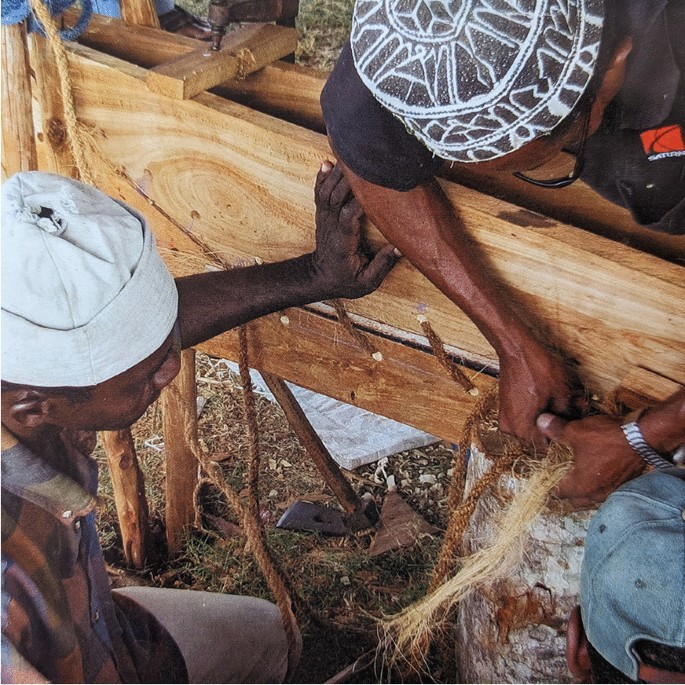In this detailed image, we observe three African-American men deeply engaged in a hands-on task involving a wooden contraption. The man at the top right, wearing a black and white patterned cap and glasses, leans over the wooden structure, meticulously tying thick ropes or twine, which resemble straw or horsehair. He is dressed in a black polo shirt featuring the Saturn logo in red and white, with a visible watch on his left wrist. To the left, another man donning a white cap and a plaid shirt steadies the wooden piece with his left hand, intently watching the actions of the first man. On the bottom right, only the blue baseball cap of a third man is visible, indicating his proximity to the group but obscuring his face. The scene is set outdoors, with dirt and grass underfoot, and an assortment of tools, including a wooden stick with a sharp metal tip, suggesting that the men might be engaged in agricultural work or woodworking. Their focused and collaborative effort illustrates a moment of dedicated manual labor.